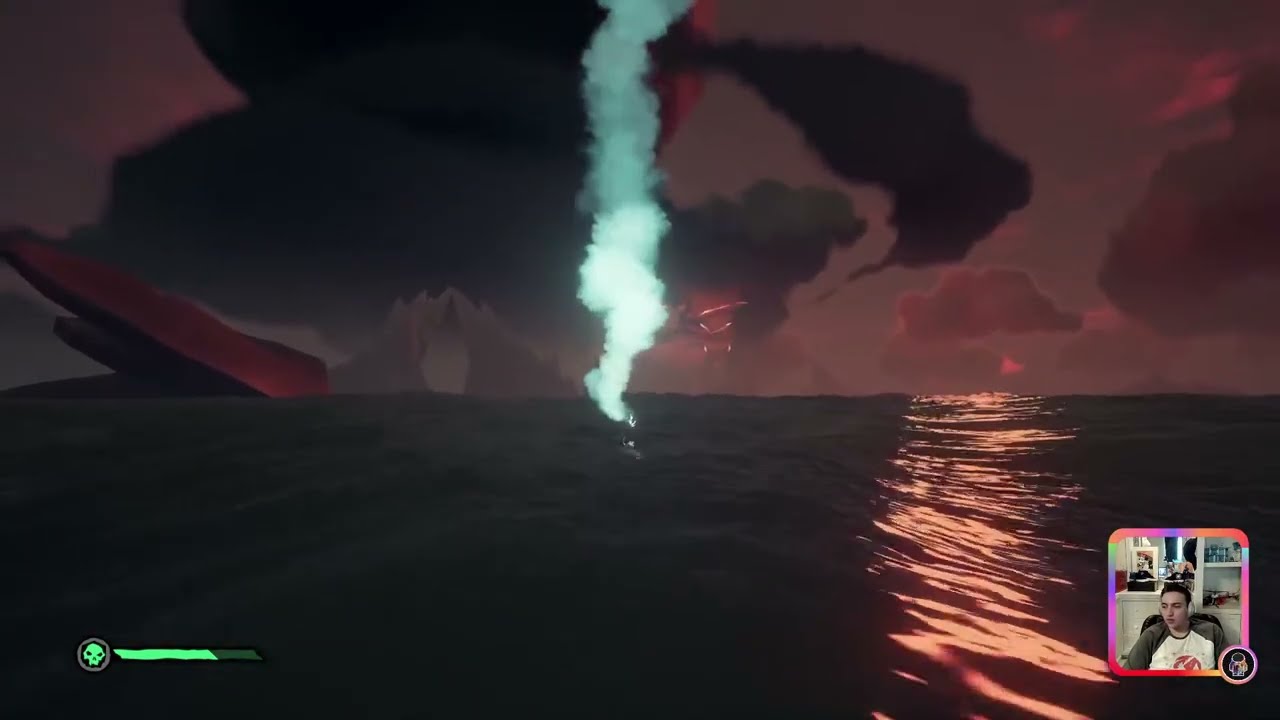The image depicts a screenshot of a video game being streamed by a player, whose webcam feed is visible in a small rounded-edge square at the bottom right corner. The streamer, wearing white headphones and a white shirt with a red logo, is seated in a room with white cupboards and a bookcase. The game screen showcases a detailed outdoor environment during sunset, featuring a vast body of water with noticeable waves. In the center, white smoke billows up from the water, suggesting a recent explosion or event. The horizon behind this scene displays dark and red-tinged clouds, providing a dramatic sky backdrop. There are rocky protrusions and islands emerging from the ocean in the background. Additionally, the game interface includes a green skull icon with a life bar located to the left, and a small animated black-and-white character at the bottom of the screen. The reflection of the moon can also be seen on the water, enhancing the visual detail of the night-time setting.